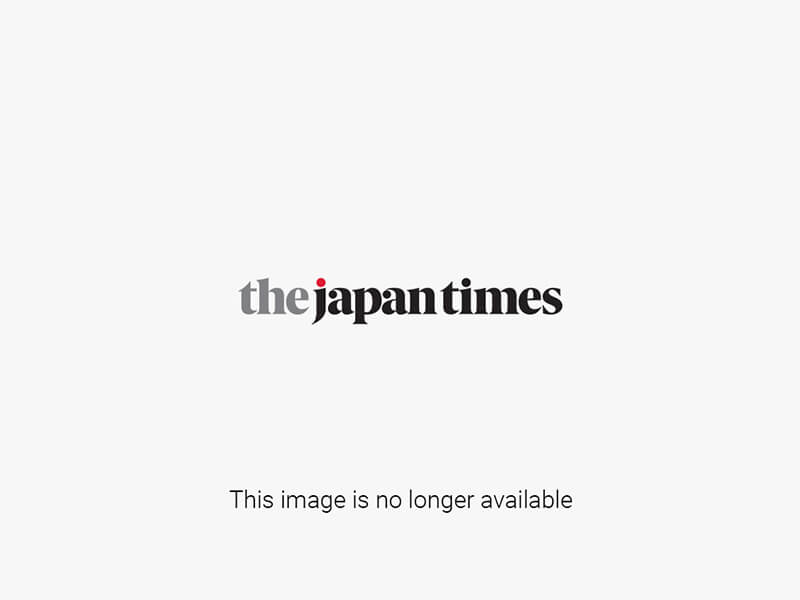In the image, a man stands slightly to the left and near the bottom of a large concrete wall, in front of an extensive painting. The man, who appears to be Asian with sparse gray hair, is dressed in a black, short-sleeved polo shirt and khaki pants that may be shorts or long pants. The concrete wall behind him holds a striking painting featuring a blue background filled with bursts of light resembling fireworks, luminescent jellyfish, or sea anemones. These bursts start with vibrant orange at the bottom and transition through shades of yellow, becoming lighter as they ascend and culminating in a bright, pure white at the top, creating the illusion of emanating light. To the right of the painting, there is a small black plaque with white text, but the fine print is too small to read.